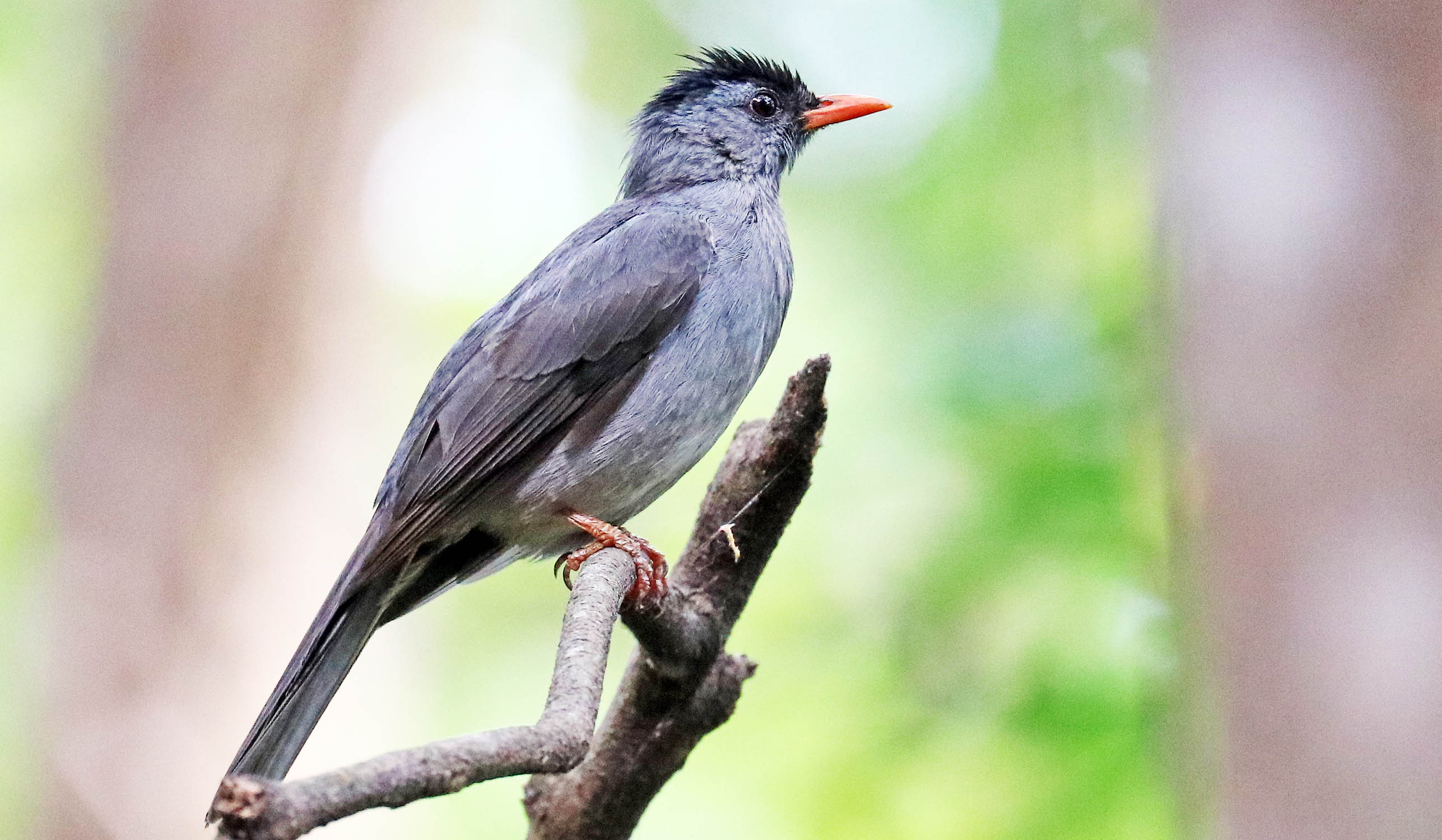This detailed image captures a small bird perched slightly off-center on a twig-like branch, facing to the right with its tail to the left. The bird is predominantly dark gray with a lighter gray breast. It sports a distinctive black crest on its head that appears similar to a mohawk, and its beak is a vivid orange, resembling a carrot. Its legs and toes are flesh-colored with black claws gripping the branch. The bird's back feathers and the tips of its wings and tail are a darker shade of gray. The background of the photograph is blurred, featuring green vegetation and indistinct, light tanned or brownish tree trunks, creating a soft contrast against the focused form of the bird.